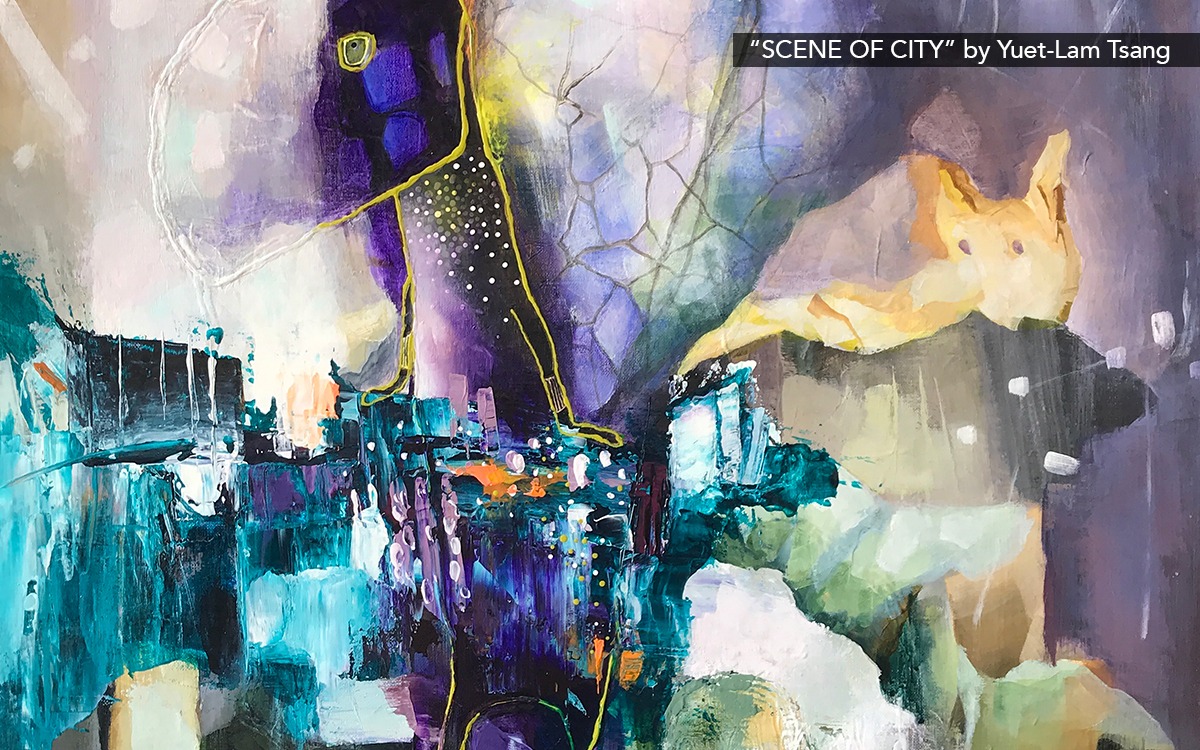This artwork, titled *Scene of City* by Yuet Lam Tsang, showcases an impressionistic and surreal cityscape rendered with a mix of deep purples, vibrant blues, pinks, aquamarine, and touches of yellow. The right side of the image prominently features a humanoid figure adorned with a headpiece resembling a bag or a mask, evoking the likeness of a pig, fox, or possibly a mouse, complemented by triangular, pointy ears. There is also a large yellow dot and what appears to be wing-like structures, suggesting veins like those of an insect. The left side is characterized by dramatic, abstract swaths of blues and purples, descending into a cascade of white dots against a backdrop of black, giving a feeling of flowing energy. The overall composition is a striking blend of abstraction and surrealism, creating a vivid and dynamic scene of a city.